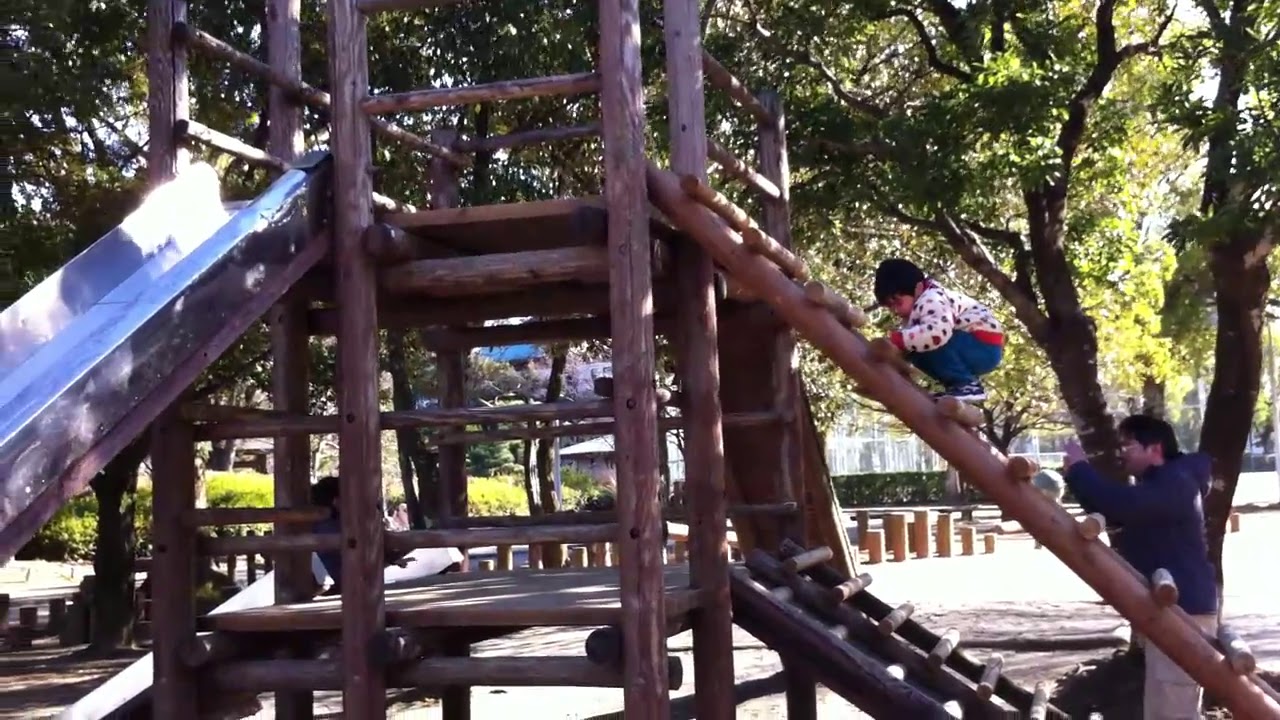In this outdoor park scene, we see a vibrant and engaging wooden playground structure resembling a small fort. The structure features various platforms and ladders with a smooth, metal chrome slide on the left side. A lower darker wooden ladder provides access to one of the platforms, while another wooden staircase climbs up to the top platform leading to the slide. At the base, a father, dressed in a blue hoodie and cargo pants, stands with his hands raised, seemingly encouraging his young son. The boy, with black hair, wears a white hoodie adorned with designs, blue pants, and gray sneakers as he climbs the ladder eagerly. Surrounding the playground, multiple trees and manicured shrubs are visible, with distant buildings and a bench accentuating the background. Circular barriers line a nearby path, all basking in the bright daylight.